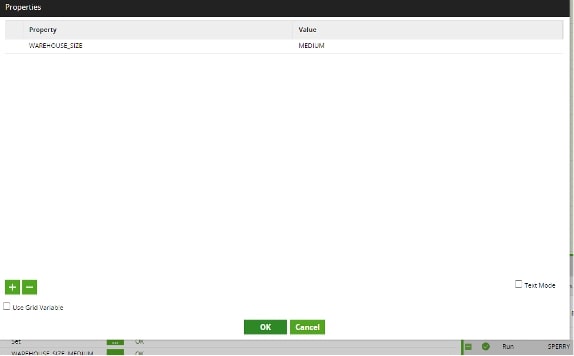The image is a screenshot predominantly filled with a white background, except for a few specific elements. At the very top, there is a thin black border stretching across the width of the image. Inside this black border, the word "Properties" is displayed in small, white, capitalized letters. Below the black border, spanning the same width but slightly shorter in height, there is a gray stripe. Within this gray stripe, the word "property" appears on the left, followed by the word "value" towards the right.

Underneath this gray stripe, the larger white area contains just one line of text. The term "WAREHOUSE_SIZE" is written in all caps on the left, with "MEDIUM" similarly capitalized on the right. A thin gray line runs from left to right beneath this line of text, creating a separation within the white background.

Moving towards the bottom-left corner of the screenshot, two small green squares are adjacent to each other. The first square features a white plus sign, while the second displays a white minus sign. Finally, on the right side near the bottom, the words "text mode" are visible.